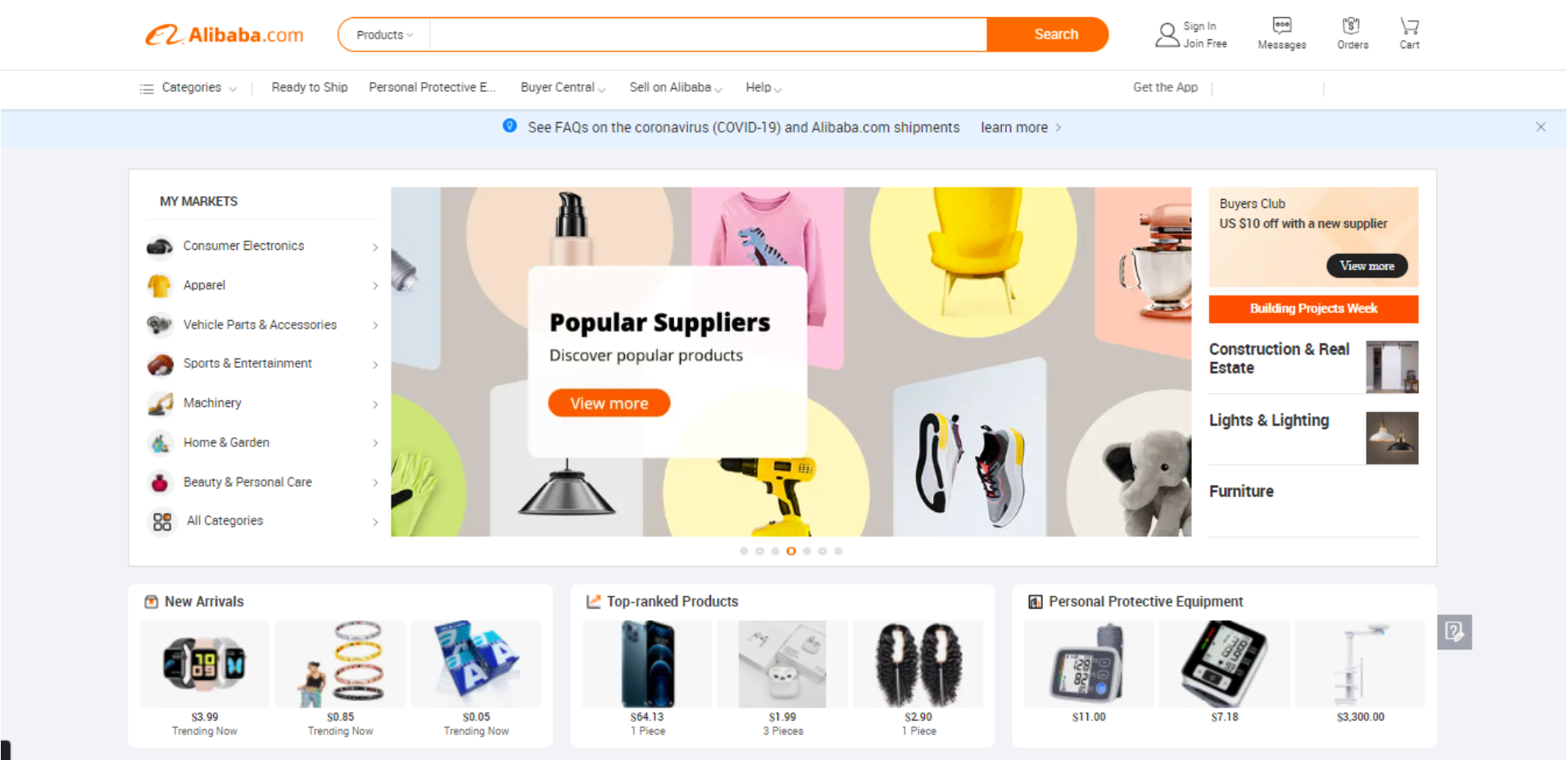This screenshot from the website alibaba.com features a bustling interface filled with various product images. At the top of the page, there's a prominent search bar for products. The assortment of items displayed includes a range of products such as makeup, a pink sweatshirt adorned with a dinosaur, a yellow chair, a kitchen mixer, a stuffed elephant, shoes, a drill, a lampshade, gloves, jewelry, watches, cell phones, wigs, and blood pressure monitors. An informational banner at the top provides a link to FAQs about the coronavirus (COVID-19) and Alibaba.com shipments. Additionally, users have the option to sign in, and there's a shopping cart icon present for easy access to purchased items.